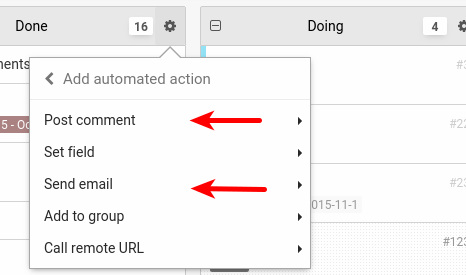The screenshot displays a website interface focused on two primary menu tiles. 

The first tile, labeled "Done," is situated on the left. Adjacent to the "Done" label is a black or gray square containing the number "16" in white. Further right, there's a gear icon, which, when clicked, reveals a detailed submenu. This submenu includes the following options:
1. **Add Automated Action**
2. **Post Comment** (with a red arrow pointing towards it)
3. **Set Field** (with a red arrow pointing towards it)
4. **Send Email** (with a red arrow pointing towards it)
5. **Add to Group**
6. **Call Remote URL**

Currently, the gear icon on this "Done" tile appears selected, as indicated by the visible submenu.

To the right, there is a second tile labeled "Doing." Next to this label is a white square displaying the number "4." Similarly, a gear icon is placed to its right; however, the specifics of its submenu are obscured by the submenu from the "Done" tile.

The image successfully captures the interactive elements of the menu interface on the website, highlighting the navigation options and the functionality provided by the gear icons.